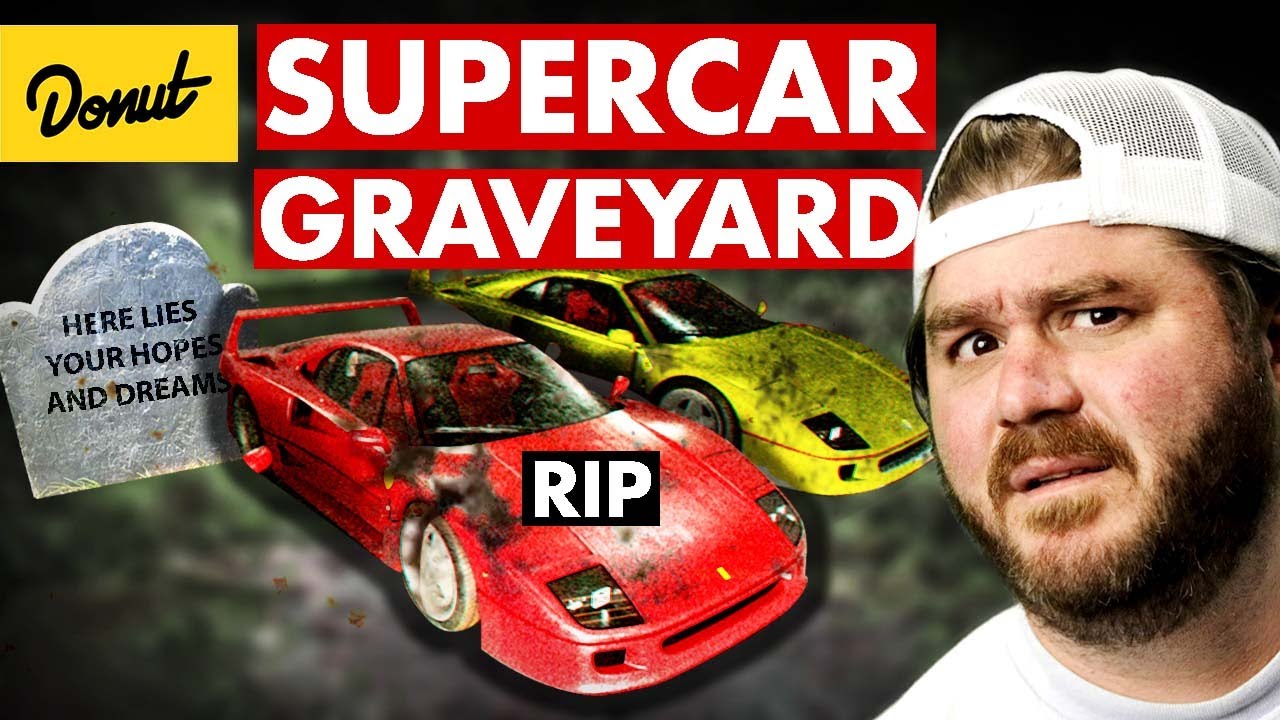In the upper left corner of the image, there is a yellow rectangle with the word "Donut" in black cursive letters. Adjacent to it are two red rectangles; the first one has "Supercar" in bold white letters, and the second, positioned below, reads "Graveyard" in similar white text. Below these signs, directly under the "Donut" label, is a tombstone inscribed with "Here Lies Your Hopes and Dreams." To its right is a red sports car featuring a rectangle on its hood that says "R.I.P." in white letters against a black background. Next to the red car is a similarly damaged and dirty yellow sports car, both showing signs of black staining and other damage effects that suggest they've been through a lot. On the right side of the image, a man with a brown beard, mustache, and brown hair peeking through a backwards white baseball cap is visible. He is wearing a white shirt and looking at the viewer with a confused or surprised expression. The background consists of blurred grass and dirt, adding to the distressed atmosphere of the scene.